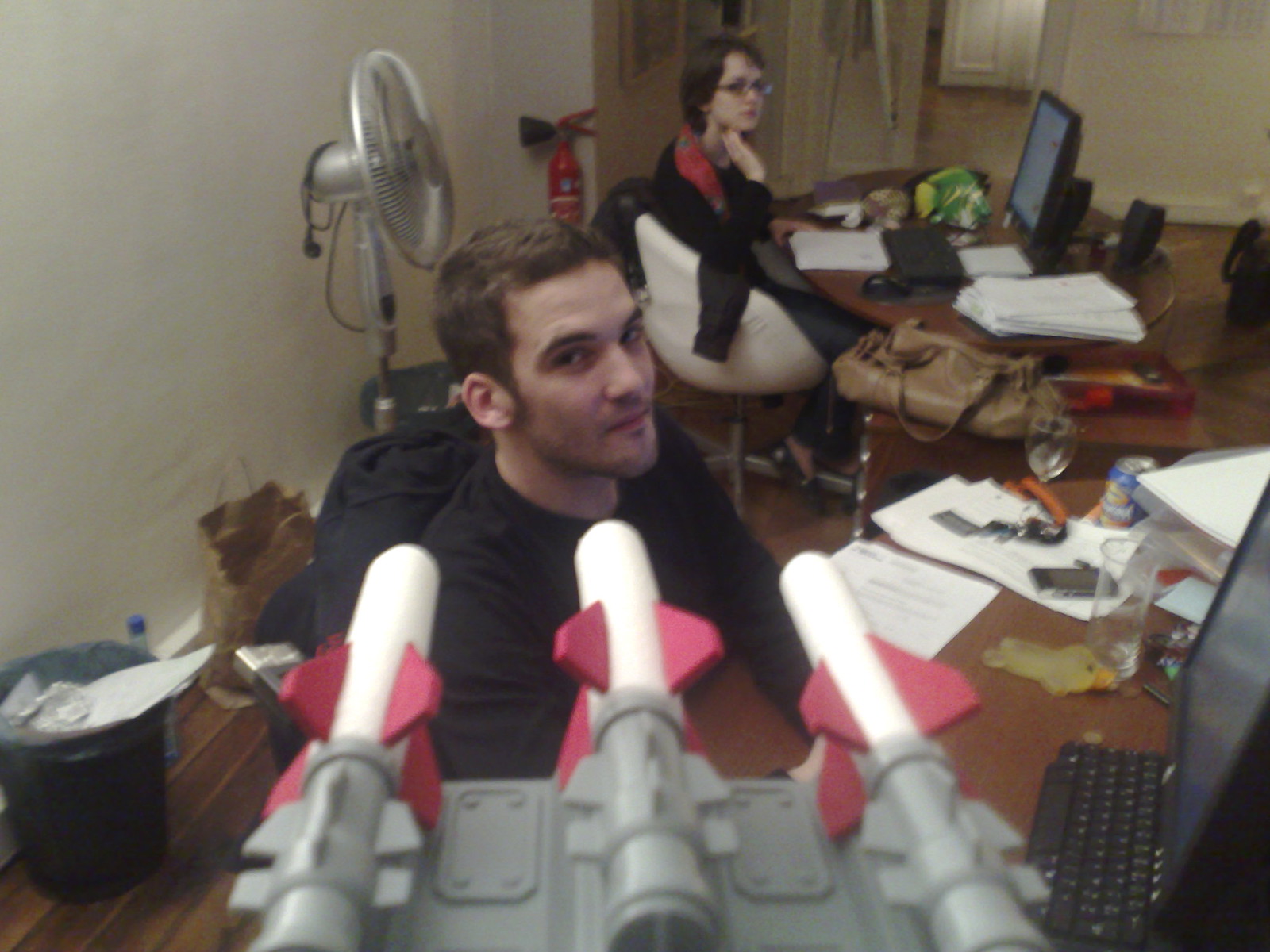The photograph captures a cluttered yet intimate indoor home office with two individuals seated at separate desks. In the foreground, a man with short brown hair, a slight mustache, and beard sits partially sideways at his desk, gazing towards the camera. Sporting a black shirt, he appears to engage with a peculiar toy or contraption—grey, white, and red—that suggests a gaming accessory, positioned close to the camera. His desk is filled with various items including a black computer monitor, keyboard, scattered papers, a glass, some keys, and other objects.

Behind him, the backdrop includes a trash can, water bottles, a brown grocery bag, and a standing fan, with a fire extinguisher mounted on the wall. At the far end of the image, a woman with brown hair and wearing glasses sits at another desk. Dressed in a black shirt and red scarf, she rests her hand on her chin. Her desk holds a computer screen, keyboard, mouse, stacks of papers, and her purse, while a jacket or sweater is draped over her chair. The overall scene portrays a functional yet disorderly workspace shared by two individuals.